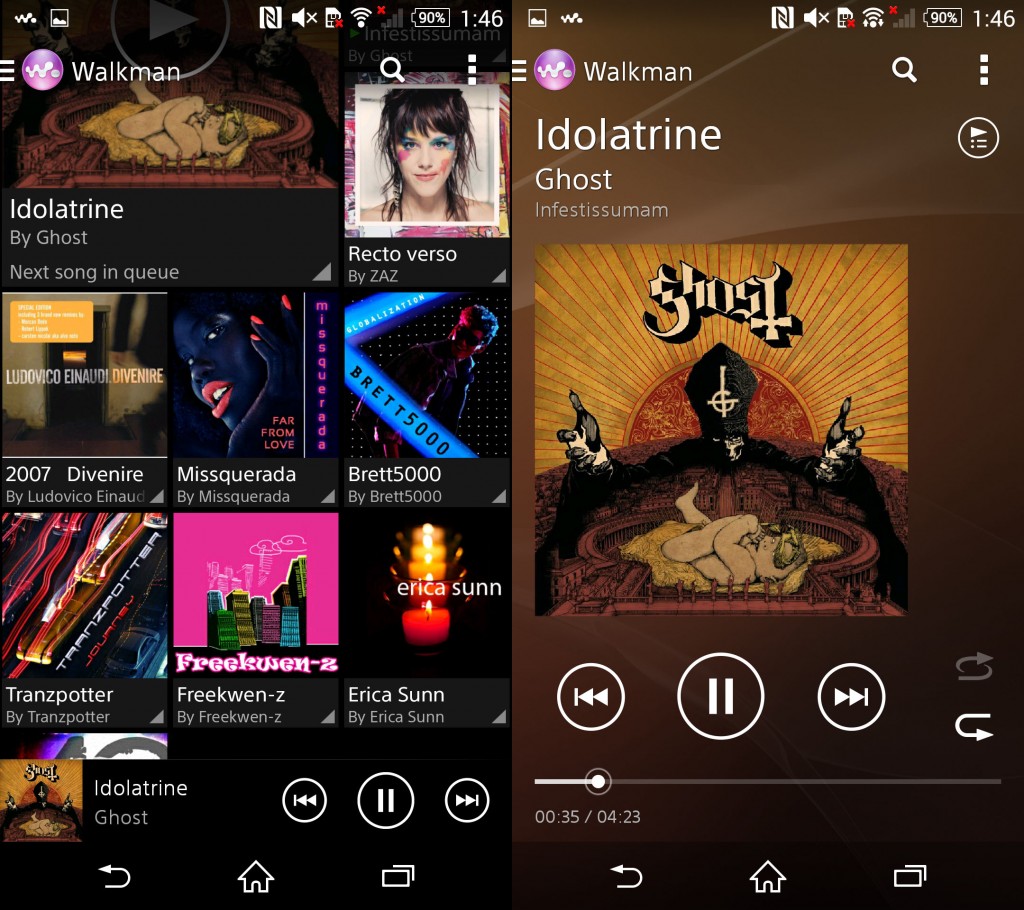The image showcases the interface of a music application resembling a Walkman, presented on two different smartphone screens.

**Left Screen:**

- **Top Section:** The top-left corner displays two icons: one is an image icon and the other appears to be the Walkman symbol. The top-right corner shows typical smartphone status icons including battery life, signal strength, and a muted sound icon.
  
- **Album and Song List:** Below the top section, there is a list of albums or songs. The currently playing album is "Adela Trine" by Ghost, with "Recto Verso" by Zaz as the next song in the queue. The list continues with the following entries:
  1. "27, Dive Nire" by Ludovico
  2. "Mascarade" by Mascarada
  3. "Brett 5000" by Brett 5000
  4. "Trans Potter" by Trans Potter
  5. "Freak Queen Z" by Freak Queen Z
  6. "Erika's Son" by Erika's Son

**Right Screen:**

- **Top Section:** The top features the Walkman logo on the left with a search bar to its right.
  
- **Now Playing Details:** Below the top section, the screen displays a blown-up view of "Adela Trine" by Ghost. The album cover is prominently shown, with the song title and artist name directly beneath it.
  
- **Control Buttons:** At the bottom, there are control buttons for rewinding, fast forwarding, and pausing the music.

This thorough depiction captures the functionality and layout of the music app across the two smartphone screens.